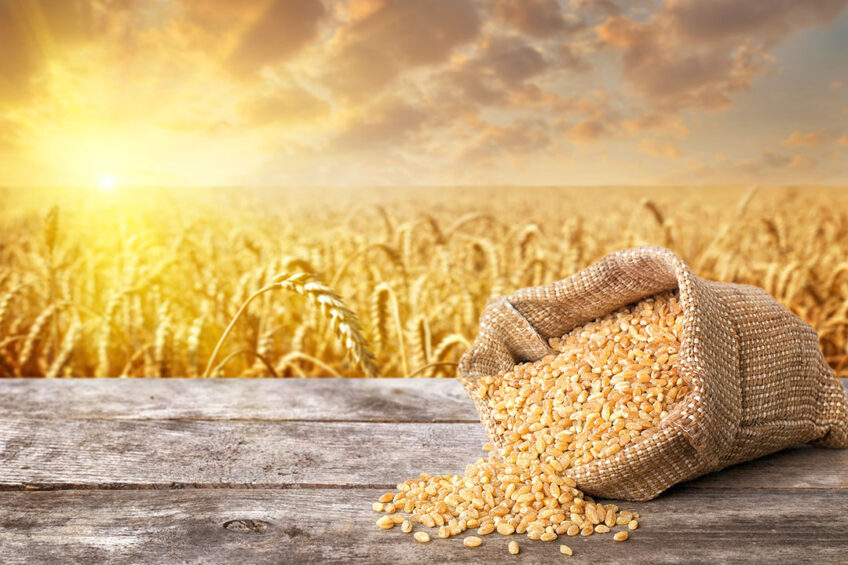In this image, we have a tranquil rural scene featuring a cloudy yet light blue sky occupying the top third of the frame, with scattered gray clouds. The sun is prominently visible in the upper left-hand portion of the image, either rising or setting, with about three-quarters of it above the horizon. Below the sky, an expansive wheat field stretches across the middle section of the image, blurring into the background as it extends. The wheat is a light brown-yellow color, capturing the quintessential look of a thriving field. In sharp contrast, the bottom part of the image is dominated by a rustic gray wooden table, detailed with visible knots and texture in the wood. Resting on this table is a brown burlap bag, which is spilling out orangish-yellow seeds or dried corn kernels. This creates a vivid foreground that complements the natural beauty of the field and sky behind it.